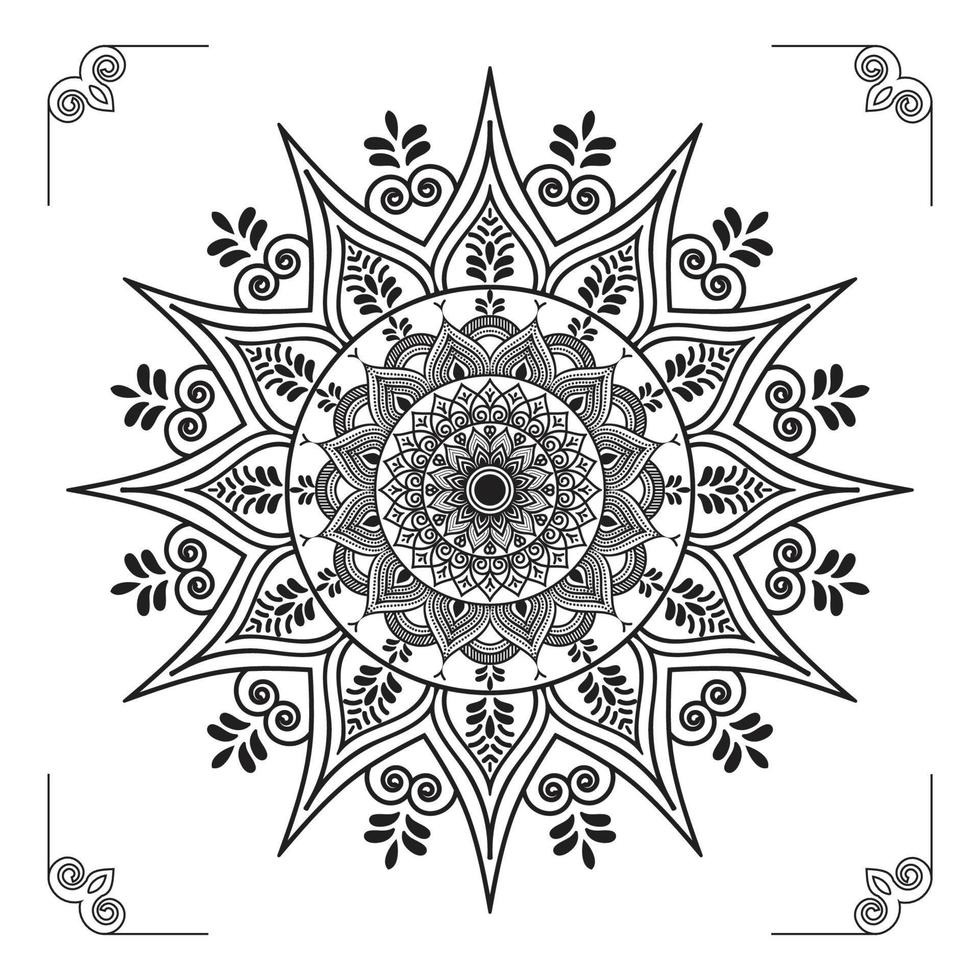This intricate black-and-white drawing resembles a mandala with a stencilized appearance, featuring crisp black line work against a white background. At the center lies a solid black circle surrounded by concentric circles, each progressively larger and adorned with elaborate patterns. The innermost circles integrate approximately 12 flares or spike-like elements that radiate 360 degrees around, some of which resemble tiny leaves or petal shapes, enhancing the symmetry and cohesion of the design.

Encasing the mandala are decorative borders with ornate caps that almost form curled edges pointing inward from each of the four corners, which add another layer of visual interest to the artwork. Overall, the piece blends symmetrical shapes—circles, flares, leaves, and teardrop forms—into a mesmerizing pattern reminiscent of a spirograph design, while also evoking traditional Indian art motifs. This detailed and harmonious composition suggests a significant investment of time and skill in its creation.